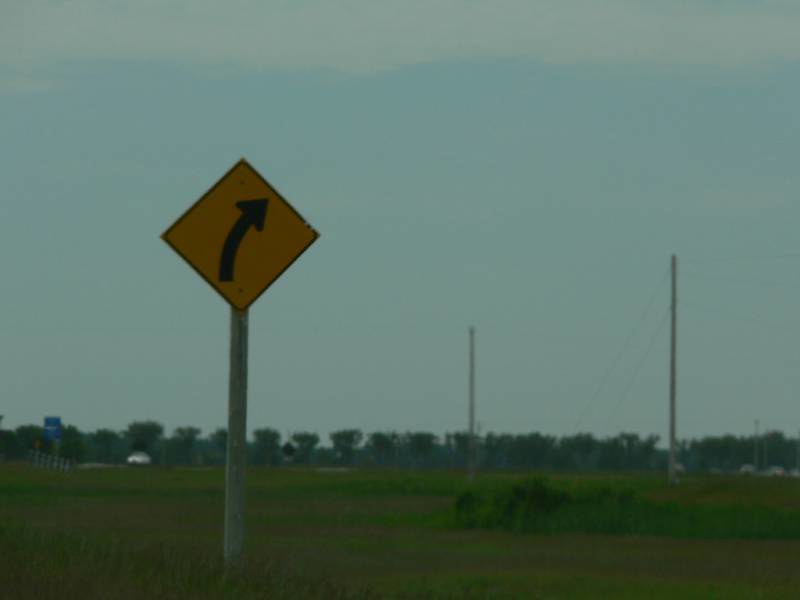This outdoor photograph captures a somewhat hazy and out-of-focus landscape on a gloomy day with blue-gray skies diffused with white clouds. Dominating the left-hand side of the image is a prominent white signpost, about a third of the way from the edge, featuring a yellow diamond-shaped road sign with a black arrow indicating a gentle right turn. The foreground displays a brown grassy field dotted with a few greens, while the mid-right section shows two power poles overshadowed by some tall bushes. Further back, we notice a uniform line of manicured trees, though mostly blurry due to the picture's lack of sharpness. Additionally, the background includes a couple of indistinct cars and a billboard on the left side, adding extra elements to the scenic yet imperfectly captured landscape.